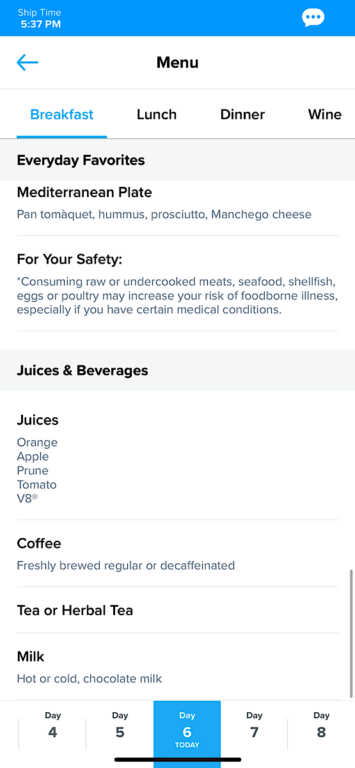The image appears to be a screenshot of a menu interface, likely from a tablet. The top section features a light blue strip with "Ship Time: 5:37 p.m." displayed on the left side and a text bubble icon on the right. Directly below this, the screen transitions to a white background with a central "Menu" heading. On the left side, a blue button is visible. 

The menu is divided into tabs for "Breakfast," "Lunch," "Dinner," and "Wine," each labeled with black text. The "Breakfast" tab is highlighted in blue, with an underline indicating it is the active selection. 

Within the "Breakfast" section, various items are listed under the heading "Everyday Favorites," featuring:

- Mediterranean Plate
- Pan tomàquet (spelled t-o-m-a-q-u-e-t)
- Hummus
- Prosciutto
- Manchego Cheese

A warning line reading, "For your safety, consuming raw or undercooked meat, seafood, shellfish, eggs, or poultry may increase your risk of foodborne illness, especially if you have certain medical conditions," follows.

Further down, a gray ribbon labeled "Juices and Beverages" separates additional sections:

- Juices: Orange, Apple, Prune, Tomato, V8
- Coffee: Freshly brewed, available in regular or decaffeinated
- Tea or Herbal Tea
- Milk: Hot or Cold, Chocolate Milk

At the bottom, there is a series of days listed (Day Four, Day Five, Day Six, Day Seven, Day Eight), with "Day Six" highlighted in blue and labeled as "Today."